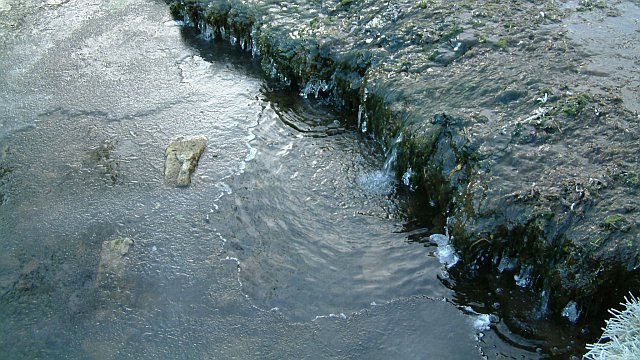The image captures a serene, winter-stream scene where a small rocky ledge serves as the focal point. Water cascades gracefully over this ledge, creating a blend of flowing and frozen elements. Atop the ledge, green moss clings tenaciously to the rocks, adding a touch of life amidst the cold. As the water falls about two feet into the creek below, it splashes and forms bubbles, indicating the motion of the clear, unpolluted water. The rocks beneath the water are visible and vary in color from tan to gray. In several places, ice has formed, some chunks still clinging to the rocks while others have fallen into the stream. The sunlight catches on the shiny ice formations, creating a mix of slick ice surfaces and areas where water continues to flow, rippling gently. The scene is harmonious, with the central flowing water breaking the stillness of the frozen surroundings and reflecting a pristine winter landscape.